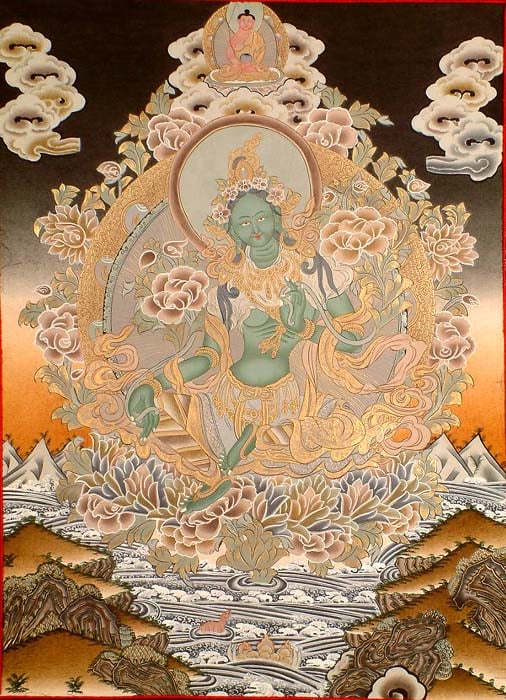This detailed painting vividly portrays a Hindu goddess with pale jade green skin, possibly one of the goddesses, seated cross-ankled in the center. Her medium braided hair is adorned with a crown of various flowers, which matches the abundant floral motifs surrounding her. She is dressed in shades of green, orange, and brown, with her right hand lifted and the left hand resting beside her. Framing her serene form is a circular halo in pale jade green tones, evoking a mirror-like frame. Above her, perched serenely amidst the clouds, is another figure resembling Buddha. The lower part of the painting portrays water, adding a tranquil element to the rich, detailed composition.